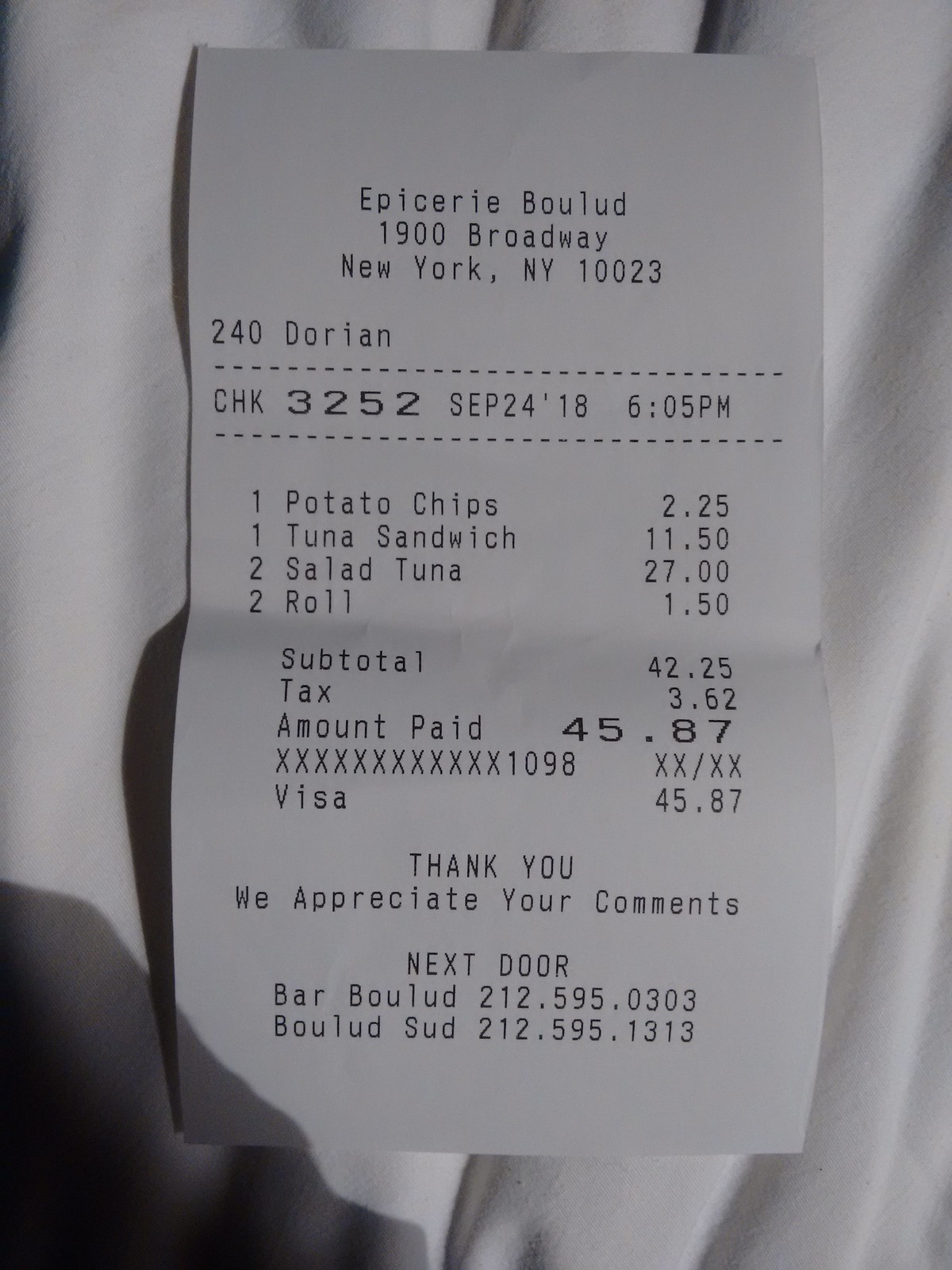Captured by a phone, the image has a portrait orientation with a greater height than width. The background is a white, rippled tablecloth or sheet, providing a textured backdrop with dark shadows accentuating the folds. A shadow, likely cast by the photographer, is visible in the bottom left corner. Dominating the center of the image is a receipt, comprising approximately 80% of the frame.

The receipt details a transaction at "Epicure, Bullard," located at 1900 Broadway, New York, 1023. The check number is 3252, dated September 24 at 6:05 p.m. The purchased items include one potato chip for $2.25, one tuna sandwich for $11.50, two salad tunas for $27.00, and two rolls for $1.50, with a subtotal of $42.25. After adding tax of $3.62, the total amount paid is $45.87, settled via Visa. The bottom of the receipt expresses gratitude with the message, "Thank you, we appreciate your comments." It also provides contact information for "Next door, Bar Bullard" (212.595.0303) and for "Bullard sued" (212.595.1313).